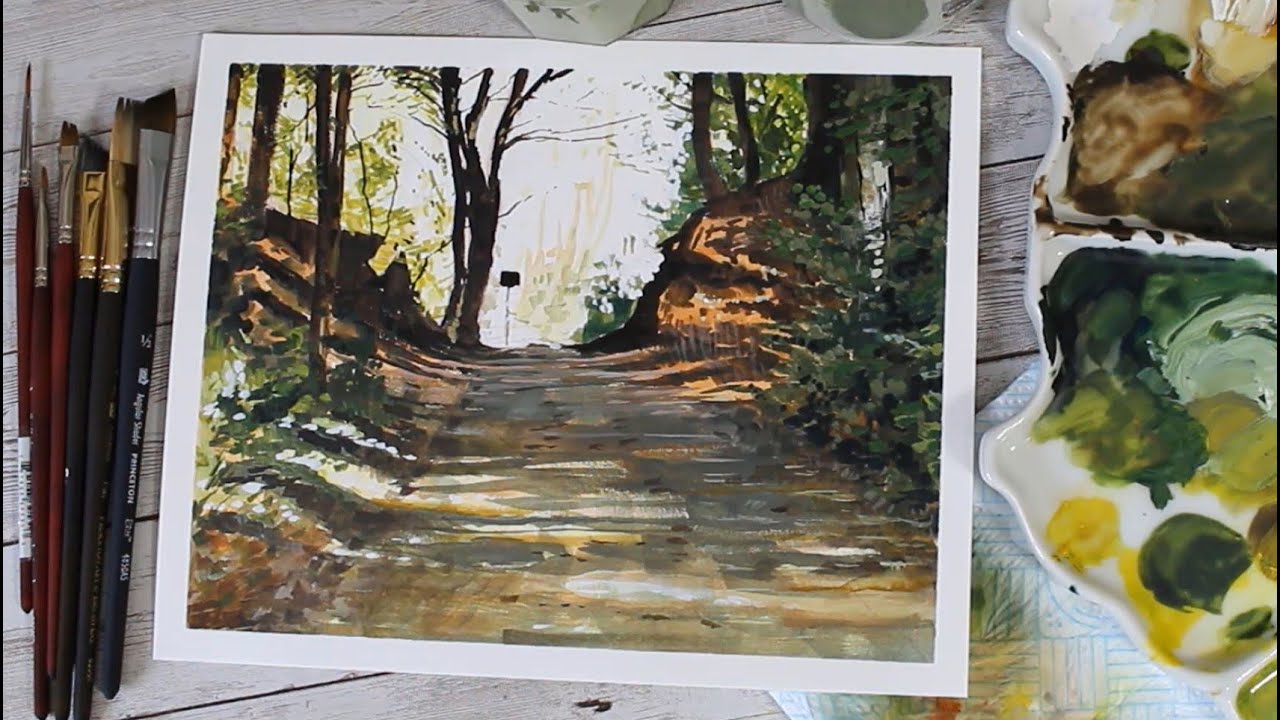This photo captures a serene woodland watercolor painting created on a rustic whitewashed wooden table with visible slats. The painting, set on a small square of paper with a white border, depicts a dirt road flanked by trees on both sides and terminating at a distant sign. The artist’s workspace surrounds the painting, showcasing their organized tools and materials. On the right side of the painting rests a white ceramic mixing dish featuring various color mixes, with earthy tones like greens, yellows, browns, and blacks. Below this dish, a folded paper towel, smudged with paint from cleaning brushes, is visible. On the left side of the painting, a collection of paintbrushes is arranged neatly—three black-handled brushes with silver and gold tips, and three brown-handled brushes of varying shapes and sizes, from medium to very fine. Slightly above the painting, there is a white ceramic cup that likely holds water for rinsing brushes. The colors used in the painting are predominantly natural earth tones, emphasizing the yellows, browns, and greens of the forest pathway, complemented by a serene white sky in the background.